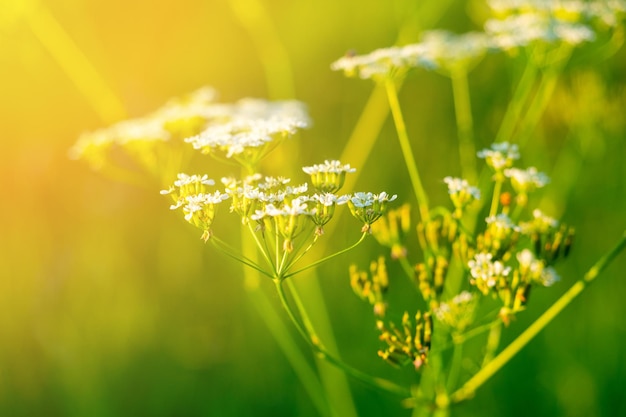In this highly detailed, up-close photograph of Queen Anne's lace, the intricate nature of the plant is highlighted with delicate, airy, teeny tiny white flowers that collectively resemble lace. The foreground features several clusters of these flowers on thin green stems, with one central flower head in sharp focus. This main cluster, composed of five to seven smaller flowers, emerges prominently slightly to the right of the center of the image. It contrasts beautifully against the otherwise blurry background. 

The photographic composition guides the eye from the focused flowers to the periphery where the image blurs into a mix of golden-yellow hues on the upper left, possibly illuminated by a soft sunbeam, to deeper greens on the bottom right. The background features more of these white flower clusters, some appearing larger yet blurred due to their distance from the focal point. Additionally, unbloomed buds and smaller green stems with yellowish tips are visible, especially on the left side, offering a richer texture to the scene. The overall effect is a dreamy, almost surreal portrait of the Queen Anne's lace flower, emphasizing its delicate and lace-like appearance amidst a softly colored and blurred surroundings.